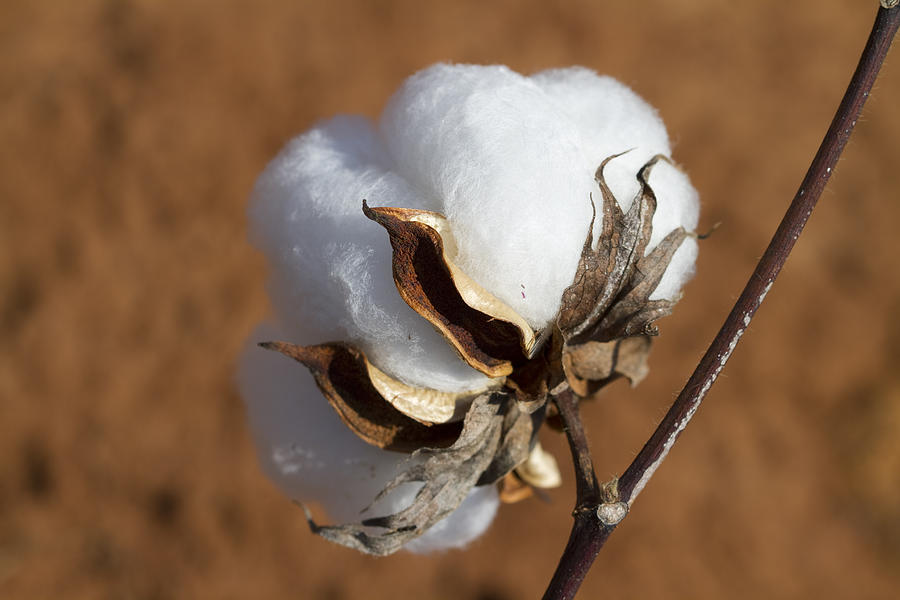In this close-up outdoor photograph, we see a cotton plant with a prominent, fluffy white cotton ball emerging from its brown stem. Surrounding the cotton ball are several wilted, orange-brown leaves. The background is blurred with a bright brownish-orange hue, likely depicting dead leaves or a dry field. This image captures the cotton in its natural growth environment, highlighting the contrast between the soft white cotton and the dying plant it sprouts from. The vivid details of the cotton ball suggest its softness and texture.